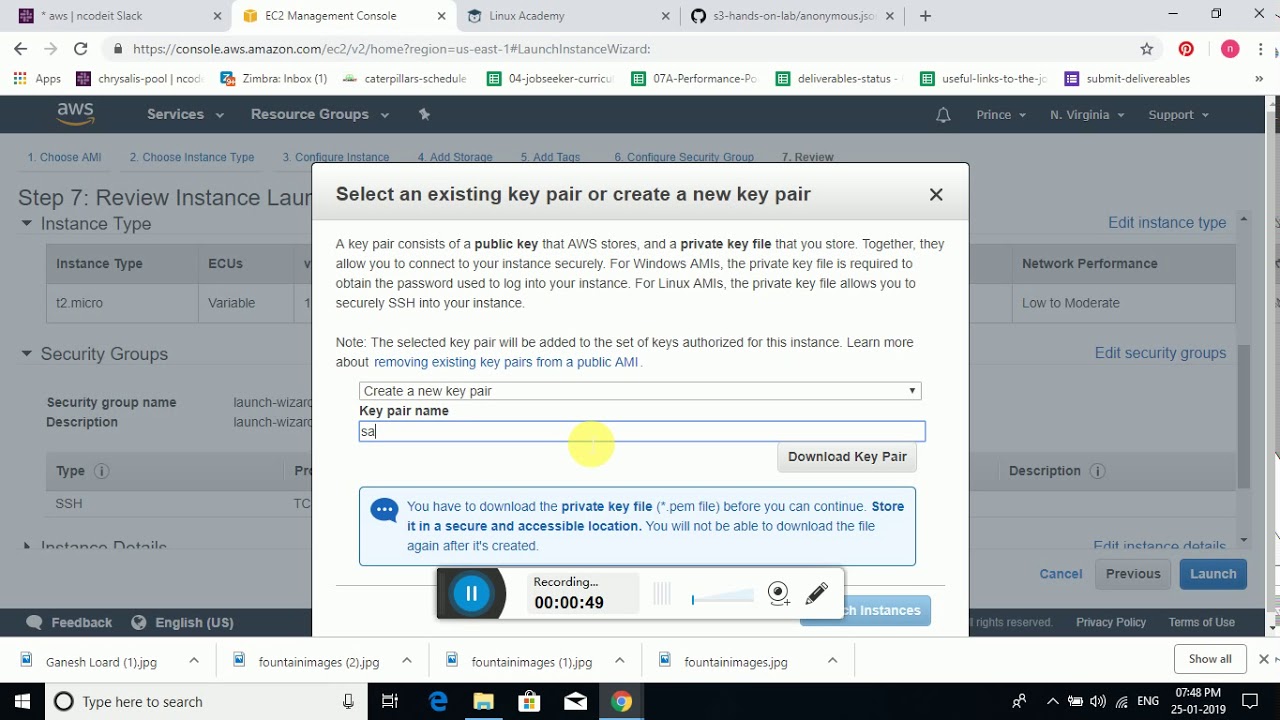This image is a screenshot of a computer screen displaying the EC2 Management Console on the AWS website. At the top of the browser window, there are multiple tabs open, but the highlighted tab reads "EC2 Management Console," indicating it is the active tab. 

Just below the tab bar, the URL displayed in the search bar is "console.aws.amazon.com," followed by additional details. The main section of the page is dominated by a rectangular dialog box with a gray header and a white body. The gray header contains the text "Select an existing key pair or create a new key pair" in black, alongside a close button (X) in the top right corner.

Within the white body of the dialog box, the user is presented with several interactive elements. The first is a drop-down menu labeled "Create a new key pair," followed by a field labeled "Key pair name" with an accompanying input box. Below this, a gray button labeled "Download key pair" invites the user to download the key pair file. Beneath this button, a blue informational box states: "You have to download the private key file before you can continue. Store it in a secure and accessible location. You will not be able to download the file again after it's created."

Towards the bottom of the screenshot, there is a small recording indicator box, featuring a circular blue button marked with a pause icon, suggesting that some form of recording or live session is currently paused.